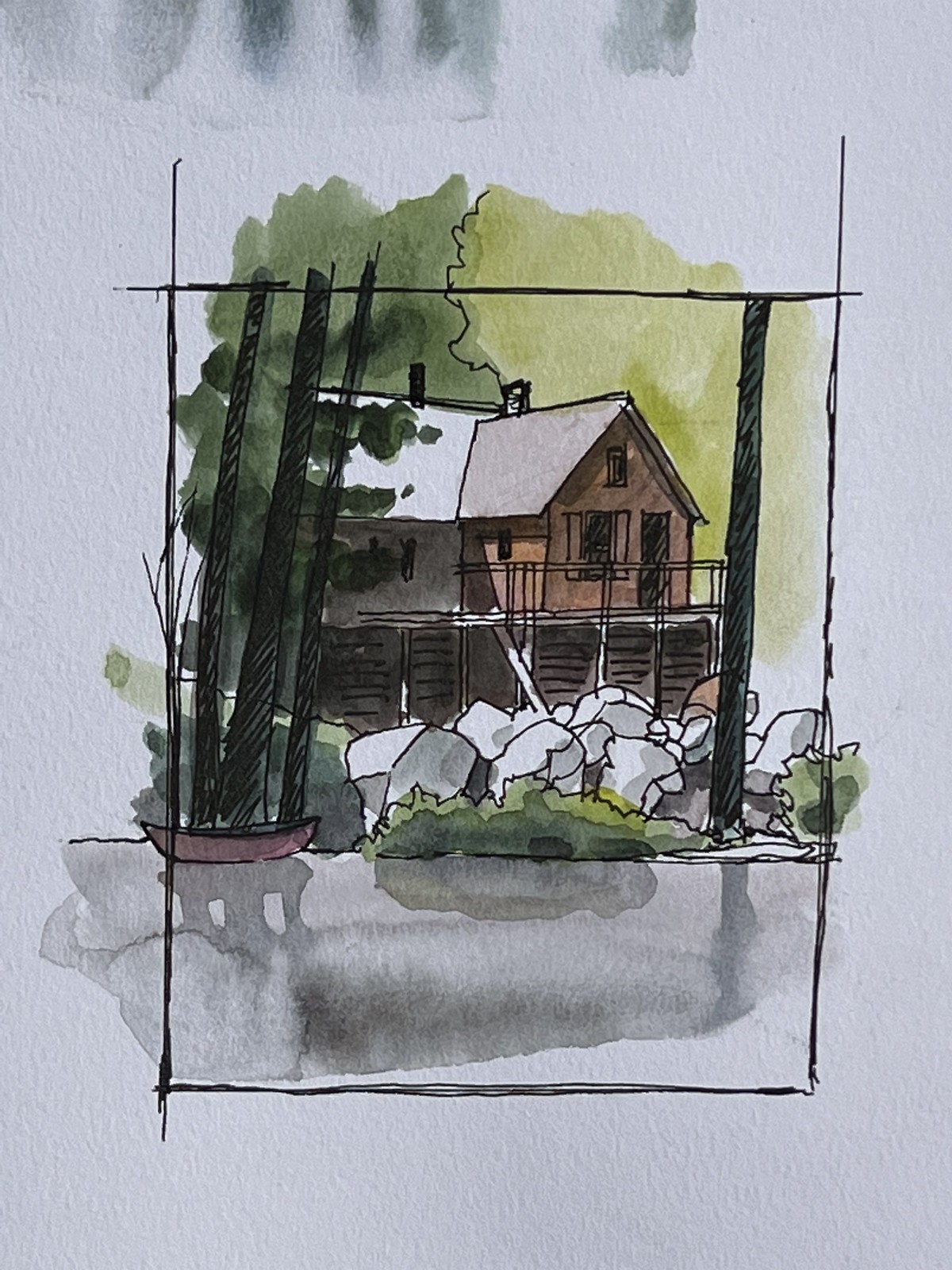This is a photograph of a watercolor painting in portrait orientation, depicting a red house with a white roof perched atop a platform or cliff, creating an elevated appearance. The house features an outdoor deck, and there is a small pot with long, oblong plants on it. The foreground includes rocks and a sprig of grass to the left, with a large tree also positioned on the left. Surrounding the house are several trees in varying shades of dark and light green. A body of water in front of the house reflects these trees, enhancing the scene with a serene quality. To the left of the image, there's a red boat on the water. The painting is framed by intersecting vertical and horizontal lines that extend slightly past their intersection, framing the scene. At the top of the painting, you can observe some characteristic watercolor paint drips, adding to its artistic charm. The overall color palette combines the earthy tones of the rocks and trees with the striking red of the house, tied together with delicate watercolor reflections at the base.